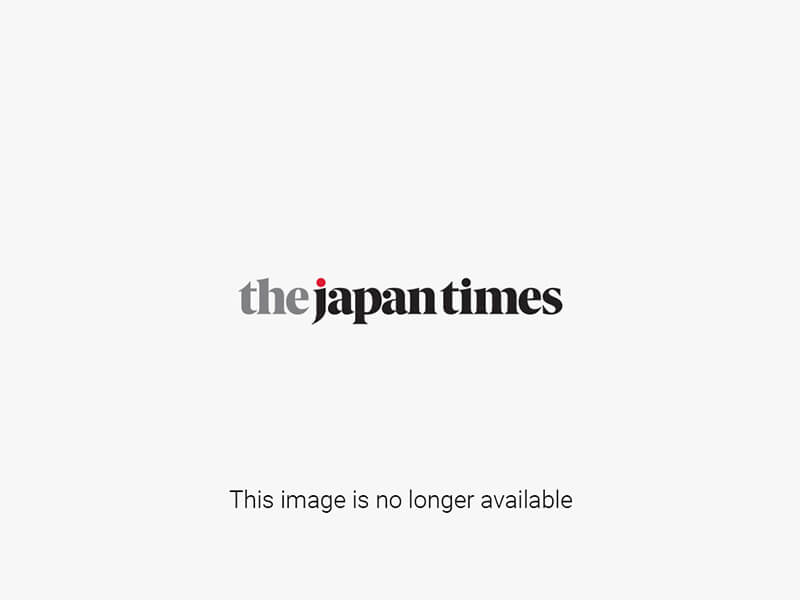The image is a detailed photograph, likely taken at a trade show or corporate exhibit in Japan, showcasing a display of automated bidet toilet seats. The display features two tiers of toilets: the first tier holding approximately five units and the second tier showcasing around ten units. Each toilet seat has a small blue plaque in front of it, presumably detailing the specifications and features. The setup is arranged neatly on a gray platform, and a large dark gray wall serves as the backdrop, adorned with white and blue Japanese text and diagrams related to the products. 

An Asian man, elegantly dressed in a black suit with black shoes and a collarless white button-down shirt, stands to the right of the display. He wears a name tag on his lapel, hinting at his official role at the event. In his left hand, he holds a clipboard or tablet, while his right hand holds a stylus or pen, which he uses to point at the toilet seats. The man, presumed to be Japanese, appears to be explaining or highlighting features to an unseen audience, reinforcing the trade show setting. A second person is partially visible in the background, adding to the bustling convention atmosphere.